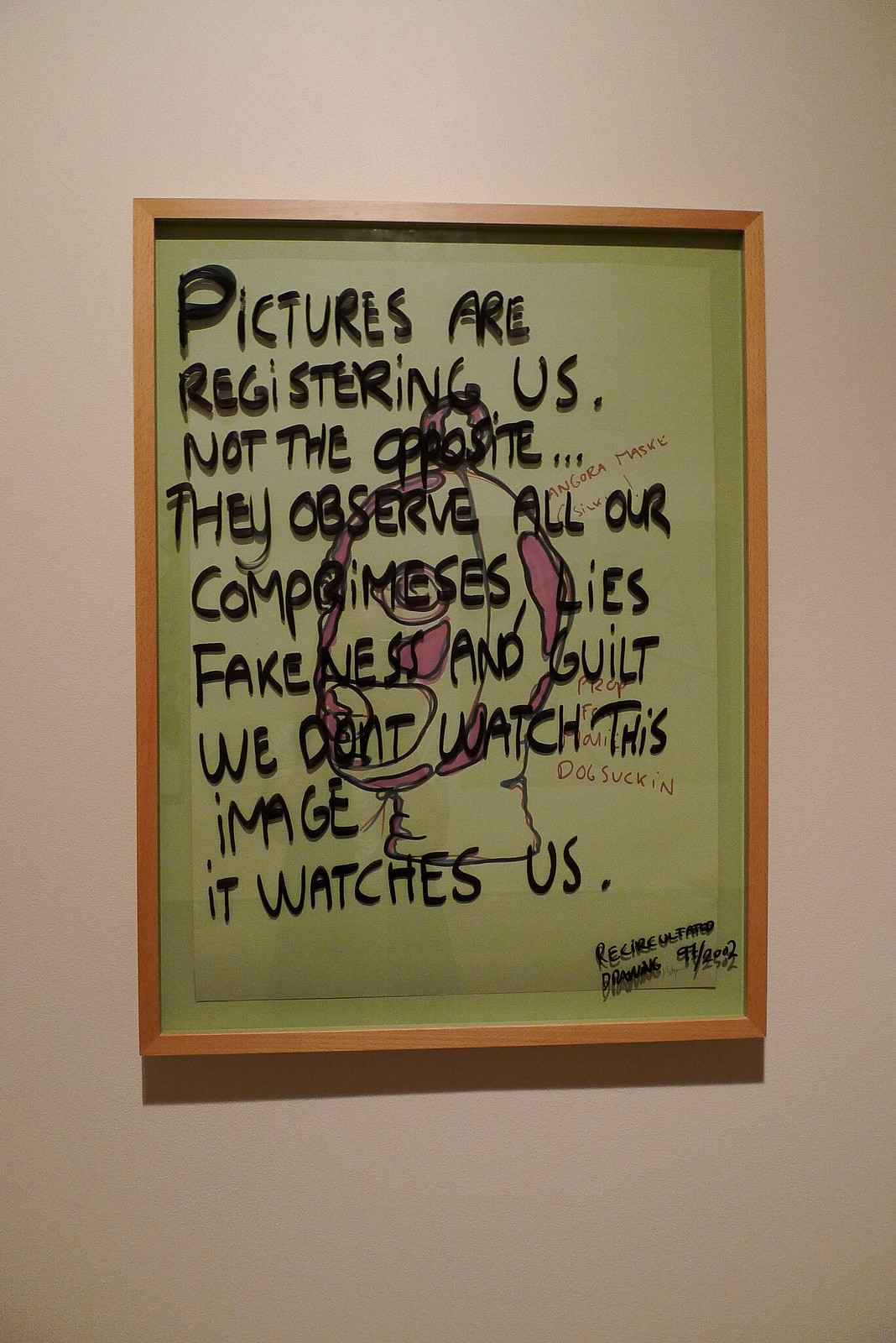This image depicts a framed artwork hanging on a completely white wall. The frame is made of a lighter wood, enclosing a picture with a solid green background. The center of the image features what appears to be a human or possibly alien face, abstract in nature, with green skin marked by purple splotches. The face, or mask, has a distinctive ball-shaped form at the top. Superimposed over this abstract art is a series of handwritten black text, which reads: "Pictures are registering us, not the opposite. They observe all our compromises, lies, fakeness, and guilt. We don't watch this image; it watches us." Written in red ink are additional annotations that are difficult to decipher. The piece is signed and dated in the bottom right corner, though the specific details are not legible. The title, "Recirculator Drawing," and the date 2002 are associated with this artwork.